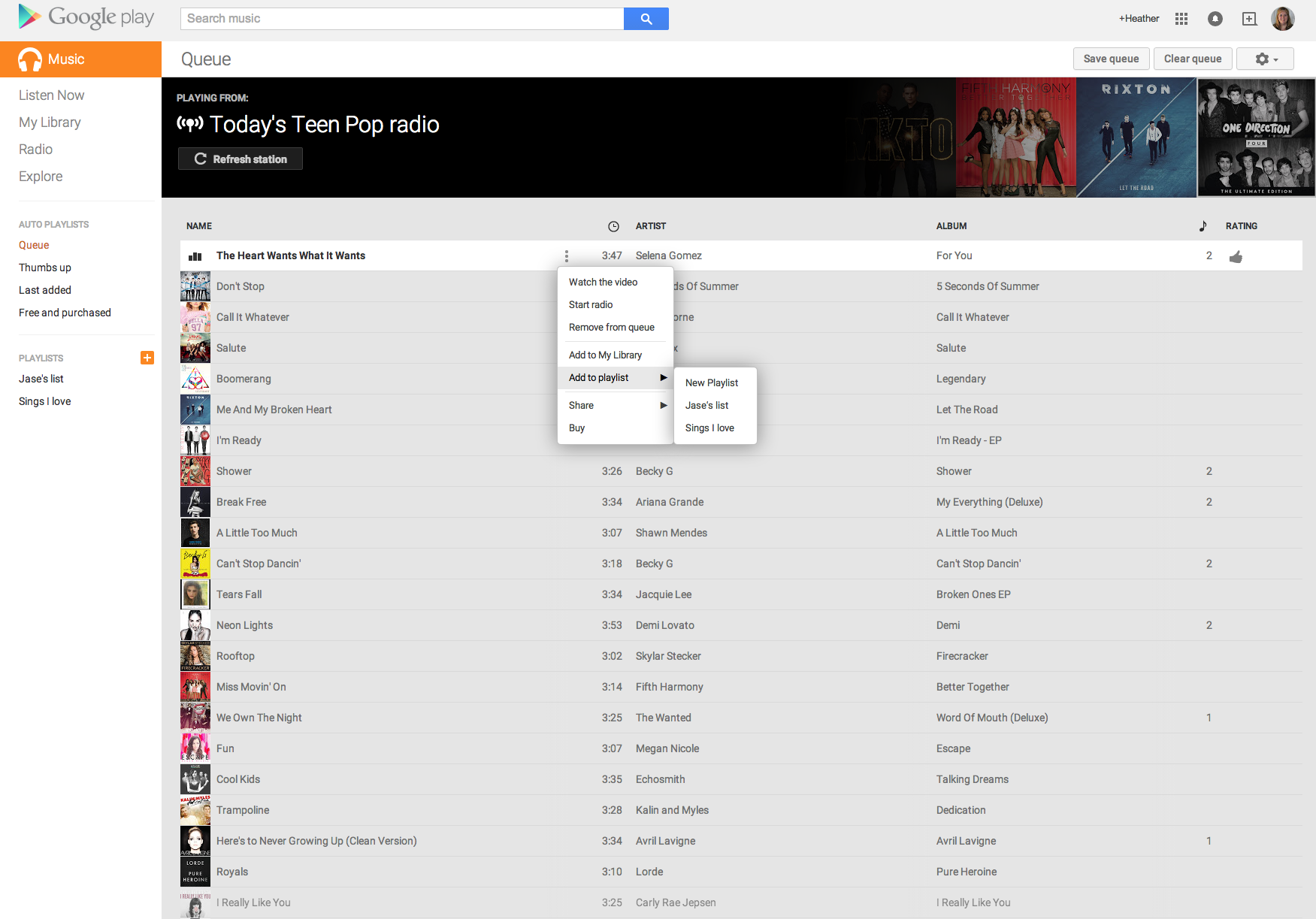In this image, we see a detailed screenshot of the Google Play interface. In the very small upper-left corner, there is the recognizable Google Play logo in a triangular shape set against a light gray header. To the right of the logo, there's a search bar with a blue magnifying glass button for search functionality. 

In the upper-right corner of the interface, the name "Heather" is displayed next to a round profile photo of Heather, which shows her face, featuring blonde hair and fair skin.

Beneath this header, a navigation bar is visible on the left side of the screen. The first item in the navigation bar is an orange box labeled "Music" in white text with a matching white icon. Listed vertically from top to bottom are several navigation options:

- "Listen Now"
- "My Library"
- "Radio"
- "Explore"
- "Auto-Playlist"
- "Cue" (highlighted in red text)
- "Thumbs Up"
- "Last Added"
- "Free and Purchased"

Beneath these options, there is a section labeled "Playlists" featuring a small orange square with a white "T" inside it. Under the "Playlists" section, two specific playlists are listed: "Jace's List" and "Songs I Love."